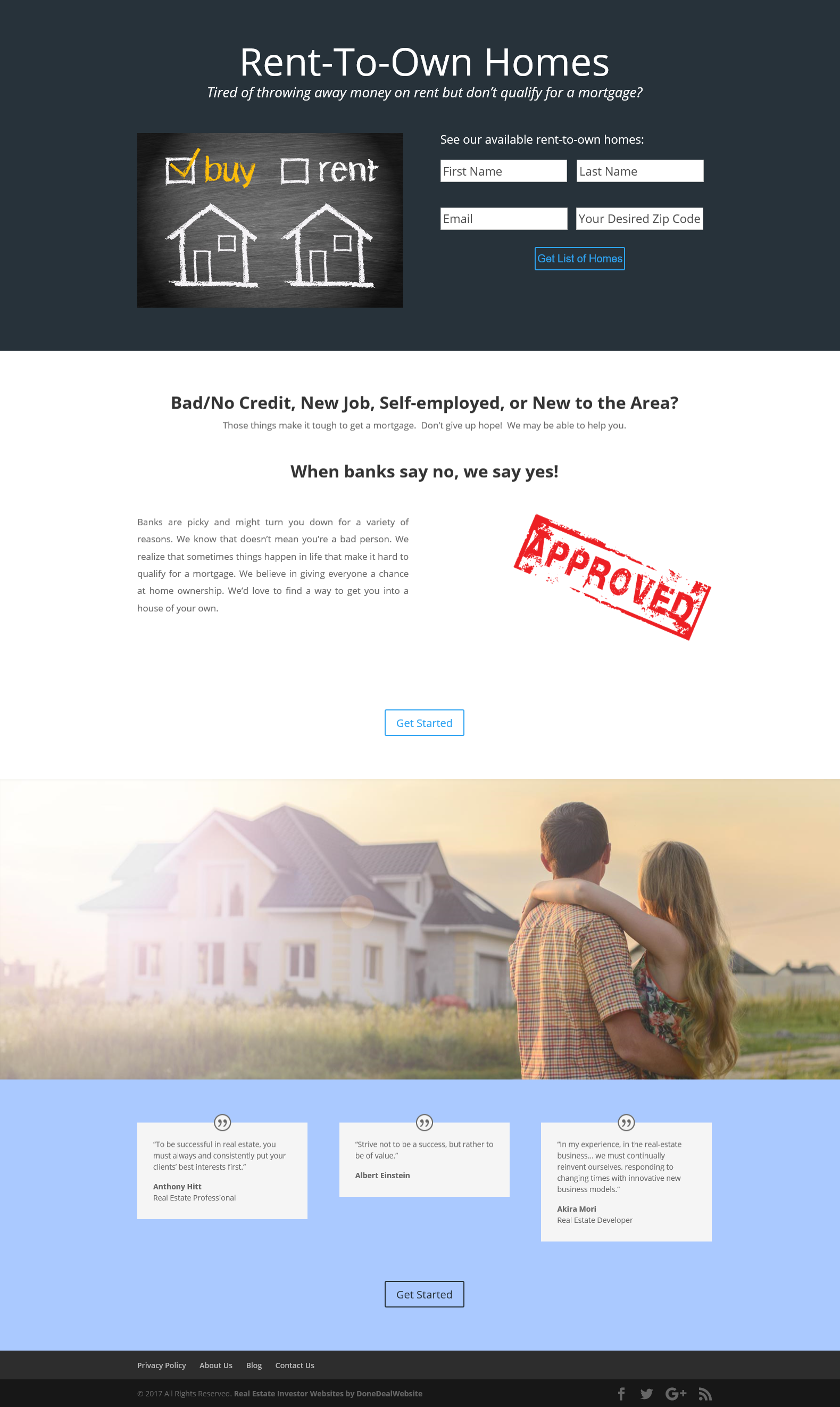This is a vertically-oriented, rectangular image designed as a promotional flyer for rent-to-own homes. The top section of the image features a navy blue, almost black background. Centered at the top, large white text reads, "Rent-To-Own Homes." Underneath this headline, in very small white font, it says, "Tired of throwing away money?" The text is so small that it is difficult to read. 

Below this, there are four horizontal white rectangular fields aligned on the right side of the page. Each field contains black text with the following labels: the first reads "First Name," the second "Last Name." Below these two, the third field is labeled "Email," and the fourth, assumed to be "Zip Code." 

Beneath these fields, there is another small blue rectangular section, though the text within it is too tiny to discern. To the left of these fields, there is a rectangular horizontal box. At the top of this box are two white squares; the first has a yellow checkmark and is labeled "buy" in lowercase letters to its right, while the second, labeled "rent," is unfilled. Below these squares are small icons of two houses.

Continuing down, in bold black font, it states, "Bad/No Credit, New Job, Self-Employed, or New to the Area?" Following this, there is smaller, unreadable black text, but then in larger, bold font, it asserts, "When banks say no, we say yes." A diagonal red "APPROVED" stamp, with its top facing the upper right corner, is prominently displayed. The word "APPROVED" is capitalized in red letters on a white background.

At the bottom of the image, there is a horizontal rectangular photograph of a real house with a green lawn. On the right side of this photograph, a couple—a man and a woman—stand with their backs to the viewer, arms around each other, looking at the house. Below this picture, a light blue section features three horizontal white rectangles with black text inside each.